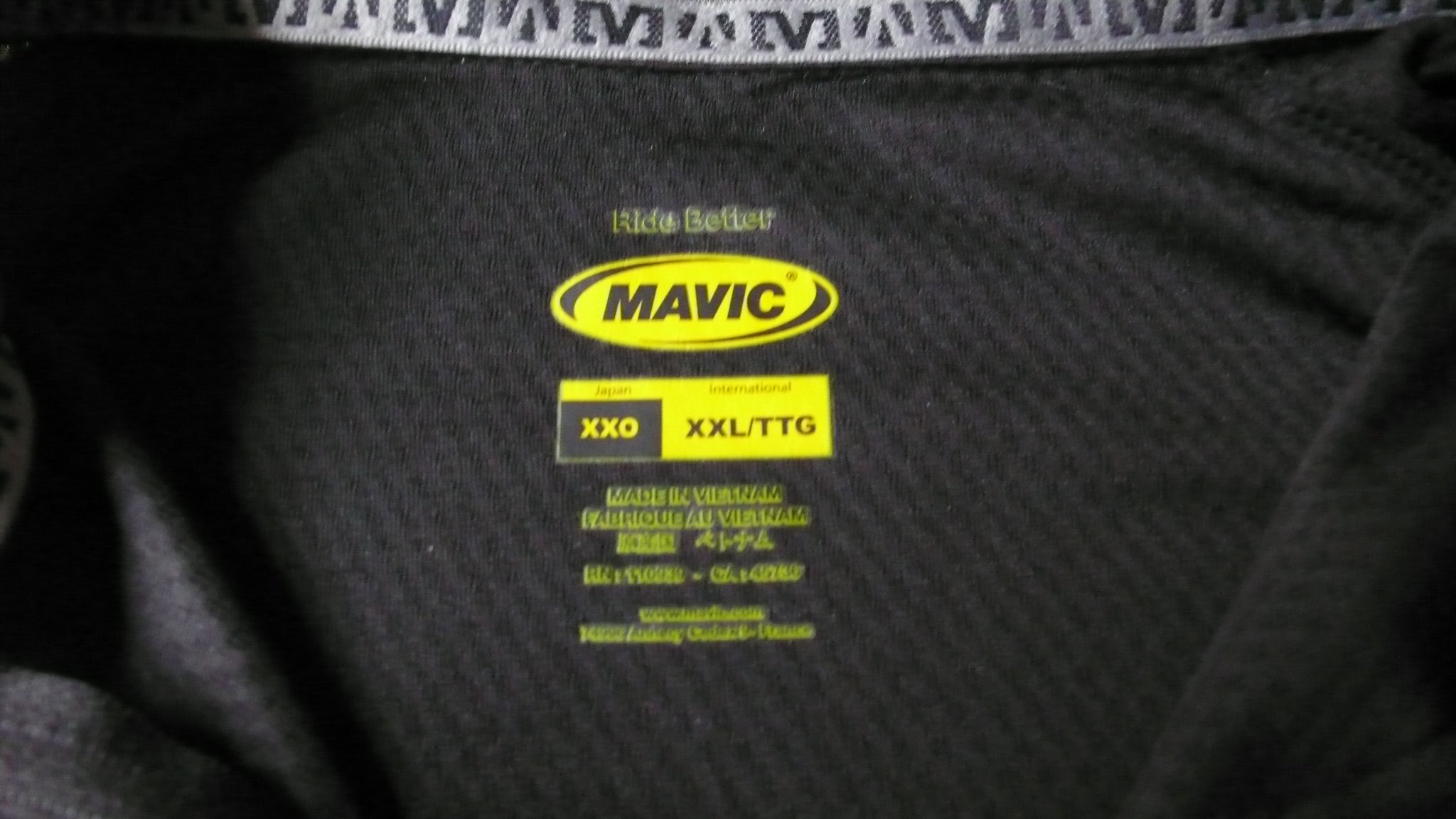The image depicts a large piece of dark gray material featuring a checkered pattern. At the top of this material is a strip of light gray fabric accented with darker gray 'M' shapes. Prominently displayed on this strip are the words "Ride Better" in bold yellow letters. In the center of the material, there is a conspicuous yellow oval with the word "Mavic" printed in gray letters. Additionally, there is an interior tag, also yellow, with a small black box in one corner displaying "XXO." Below this, in black text, it reads "XXL/TTG," followed by detailed information about the material's composition and care instructions.